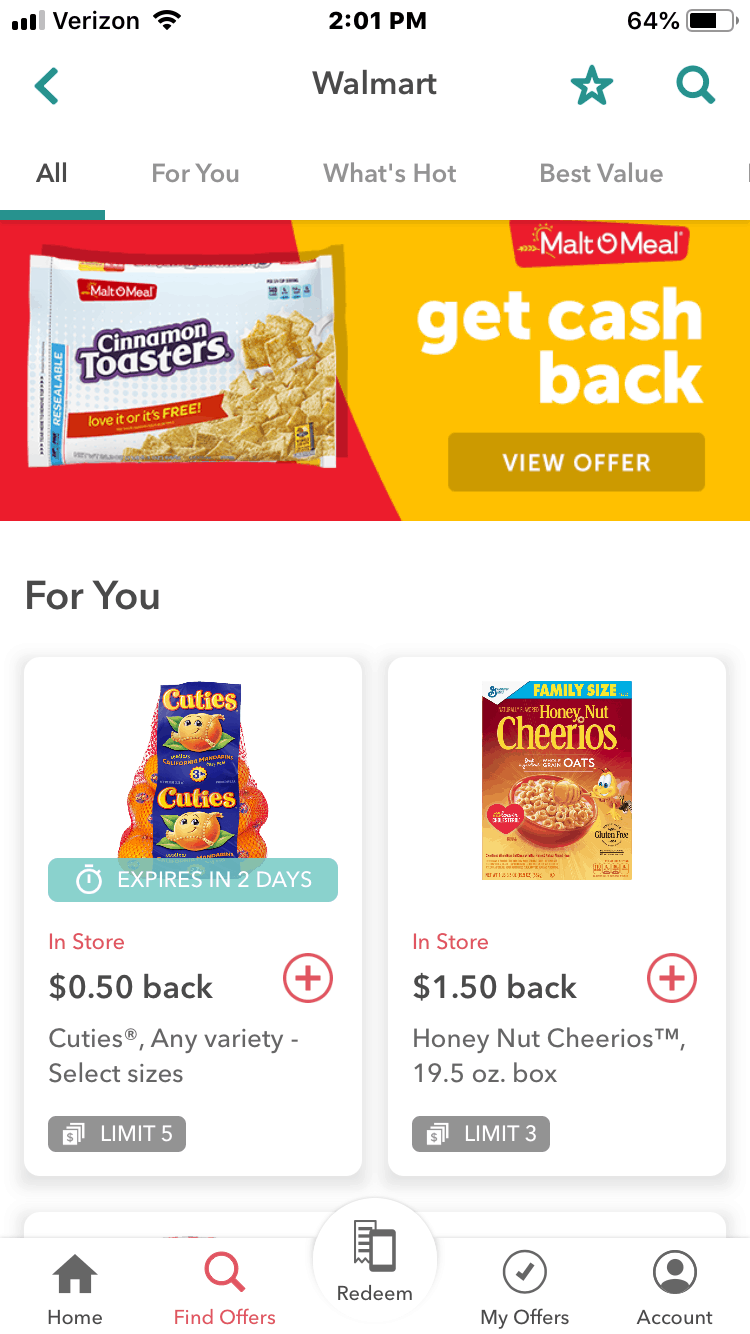Here is a detailed and cleaned-up descriptive caption for the image:

---

The image showcases a mobile phone displaying the Walmart app interface. At the top of the screen, the status bar indicates the time as 2:01 PM and the battery life at 64%. The app's header prominently features the Walmart name, flanked on the right by a green star and a green magnifying glass icon.

Directly beneath the header, four navigation tabs are visible, labeled as "All," "For You," "What's Hot," and "Best Value." The main content area begins with a brightly-colored banner advertisement for Malt-O-Meal's Cinnamon Toasters cereal on the left side, accompanied by a "Get Cash Back" text and a "View Offer" button on the right side.

The "For You" section follows the banner, displaying two featured items side by side. On the left is a stock photo of Cuties tangerines, adorned with a translucent green tag indicating an expiration in two days. Below the photo, an "In-store 50% Cash Back" offer is mentioned, including a limit of five items, with a red plus sign next to the price.

To the right is a Cheerios Family Size box, specifying the Honey Nut Cheerios 19.5 ounces variant. The offer details an in-store cash back of $1.50, a red plus sign next to the price, and a gray tag indicating a limit of three items.

At the bottom of the mobile screen, a navigation bar includes icons labeled "Home," "Find Offers" (highlighted in red), "Redeem," "My Offers," and "Account."

---

This detailed caption provides a comprehensive overview of the image and the app's interface, ensuring a clear understanding for anyone reading it.